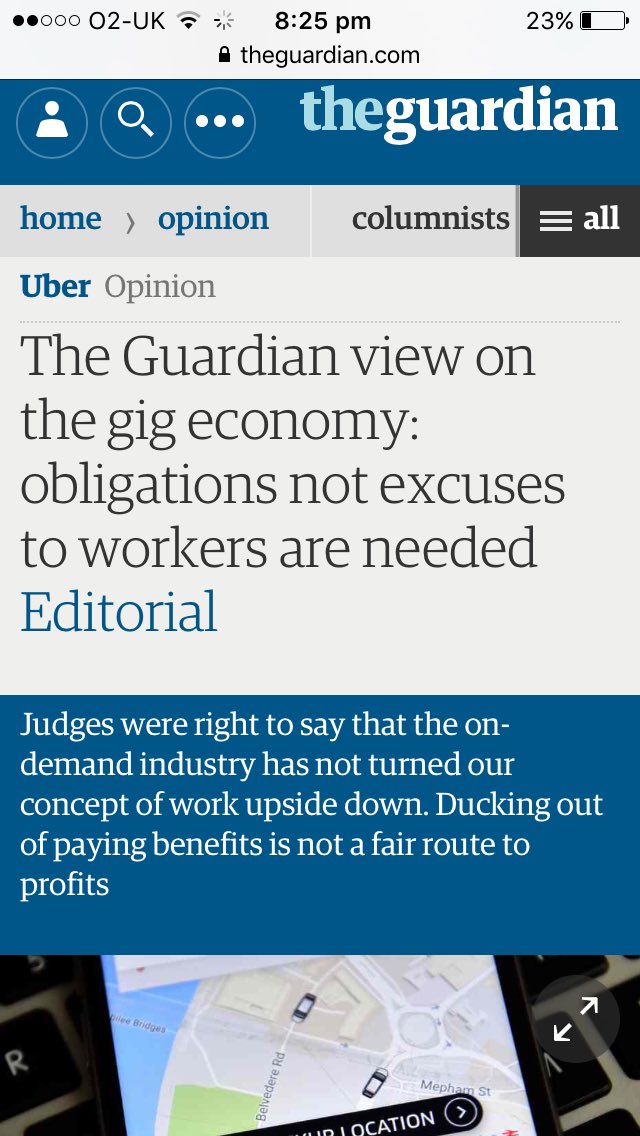**Screenshot of a Mobile Browser Showing The Guardian Article on Gig Economy**

The screenshot captures the screen of a smartphone with a background gradient that transitions from gray to blue. At the top of the screen, the status bar displays several icons, including signal strength and Wi-Fi indicators. Two specific icons are highlighted, and the text "02-UK" denotes the network provider. The status bar also shows the current time as 8:25 p.m. and a battery level at 23%, accompanied by a lock symbol. The web address "theguardian.com" is prominently featured.

Beneath the status bar are three icons representing a person, a search function, and a menu with three dots. To the right, "The Guardian" is displayed, with "THE" in light blue and "Guardian" in white. Below this, navigation options are listed: "Home," followed by a caret pointing right, "Opinion," and "Columnists." The "All" tab is currently highlighted.

The main content begins with a section titled "Uber Opinion," followed by a dotted line. The main headline reads, "The Guardian view on the gig economy: obligations, not excuses, to workers are needed," tagged as an editorial in blue. A blue bar section contains white text stating, "Judges were right to say that the on-demand industry has not turned our concept of work upside down. Ducking out of paying benefits is not a fair route to profits."

At the bottom portion of the screenshot, there is an image depicting a small section of a keyboard with a smartphone resting on top of it. The phone's screen shows a map, though only a small part of both the keyboard and the phone is visible.